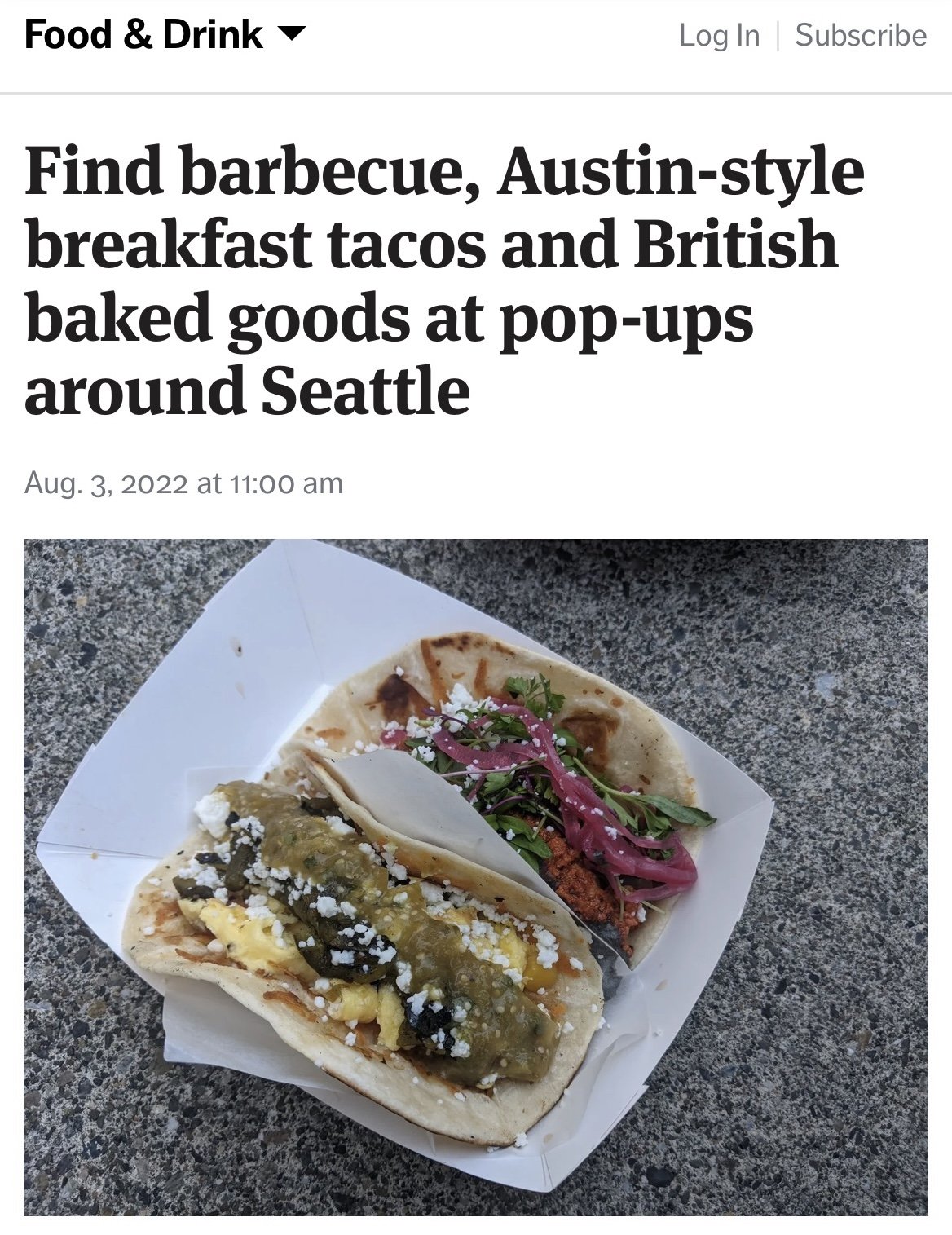The image depicts a flavorful photograph featured in a web article. The article, titled "Find Barbecue, Austin-Style Breakfast Tacos and British Baked Goods at Pop-Ups Around Seattle," is dated August 3rd, 2020, at 11 AM, and is categorized under "Food and Drink." The page also includes "Log In" and "Subscribe" options in the upper right corner. The focal point of the image is a white container holding two distinctive street tacos, set against a black and gray speckled marble countertop. One taco showcases scrambled eggs, melted cheese, and a splash of green salsa, while the other is filled with barbecued beef, onions, and fresh greens. The white tortilla shells house vibrant colors and ingredients, highlighting the unique fusion of Austin-style breakfast elements in what appear to be non-traditional tacos.